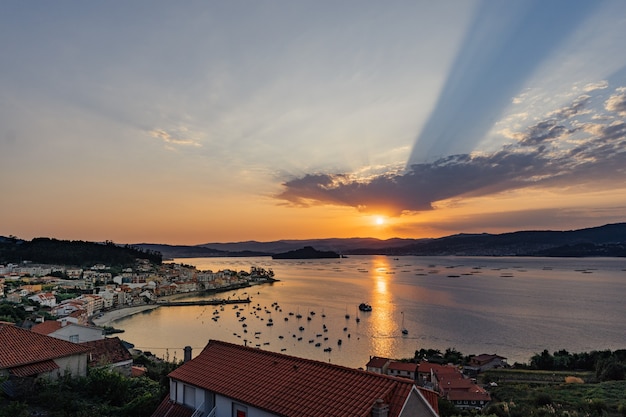This image captures a breathtaking aerial view of a serene, picturesque coastal town at sunset. The expansive scene showcases a large body of water that could be a substantial lake or bay, surrounded by majestic mountains on the horizon. The tranquil water is dotted with numerous boats, suggesting a bustling harbor or fishing activity returning at dusk. The town, characterized by its quaint Mediterranean-style architecture, features clusters of houses with iconic orange terracotta roofs and off-white walls, tightly nestled along the coastline. The coastline itself is adorned with a plethora of trees and a small pier stretching into the water. Above, the sky is painted with the striking hues of an amber sunset, interspersed with patches of gentle clouds, blending beautifully with the remaining blue of the day, casting an ethereal glow over the entire landscape.